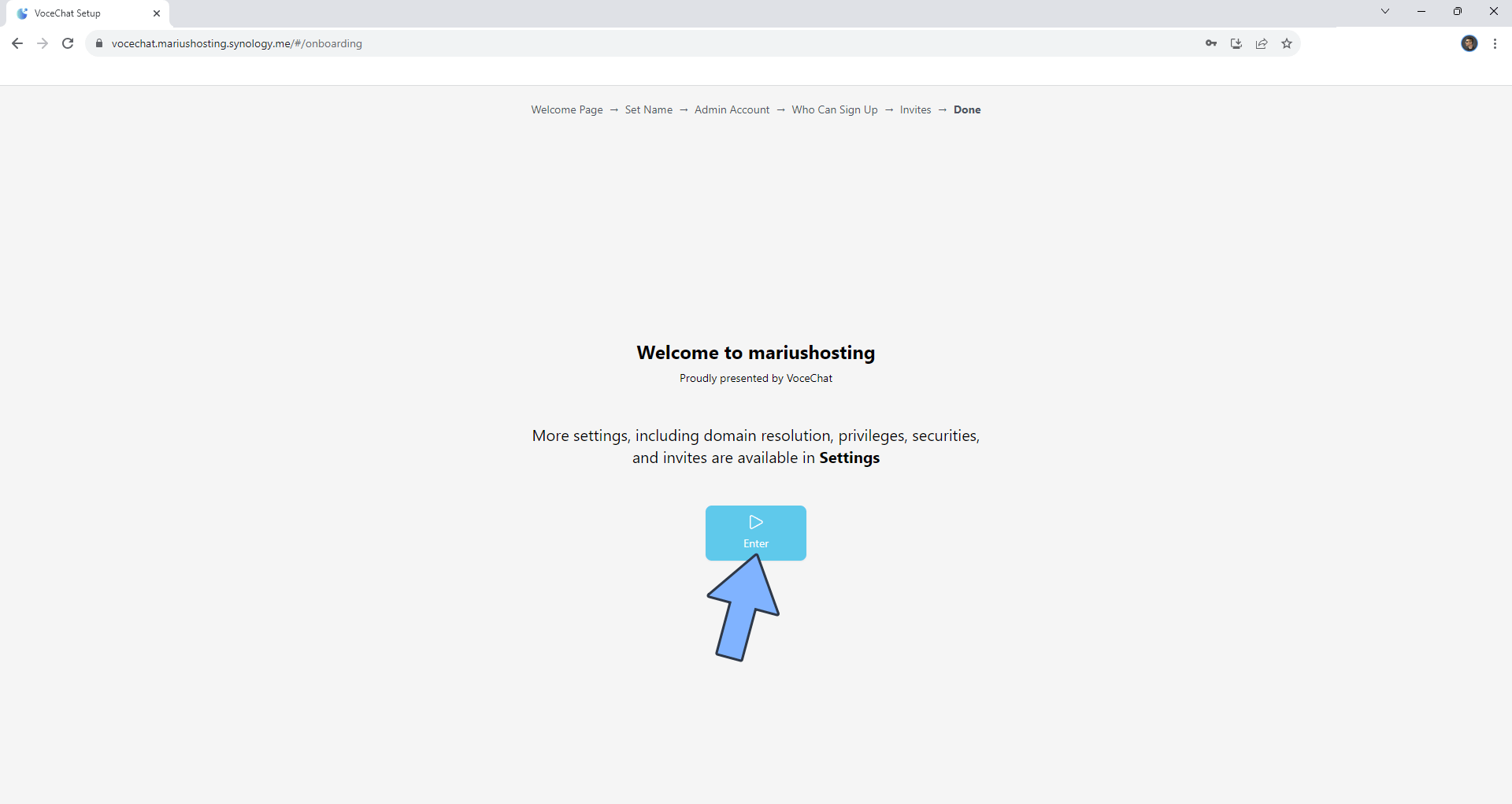This image shows a screenshot from a website, depicting a voice chat setup. At the very top of the image, a browser tab reads "Voice Chat Setup." The webpage itself features a light gray and white color scheme. In the top center of the page, there is text listing various options: "Welcome Page," "Set Name," "Admin Account," "Who Can Sign Up," "Invites," and "Done."

Below this section, in large, bold black letters, the text says, "Welcome to Marius Hosting. M-A-R-I-U-S hosting proudly presented by VOCE chat." Following this, there is a note highlighting additional settings: "More settings including domain resolution, privileges, securities, and invites are available in settings." The word "settings" is also in bold black letters for emphasis.

Further down, a blue rectangular box features a white play button at its top. Inside the box, the word "Enter" is displayed at the bottom in white text, accompanied by a sky blue arrow pointing towards it.